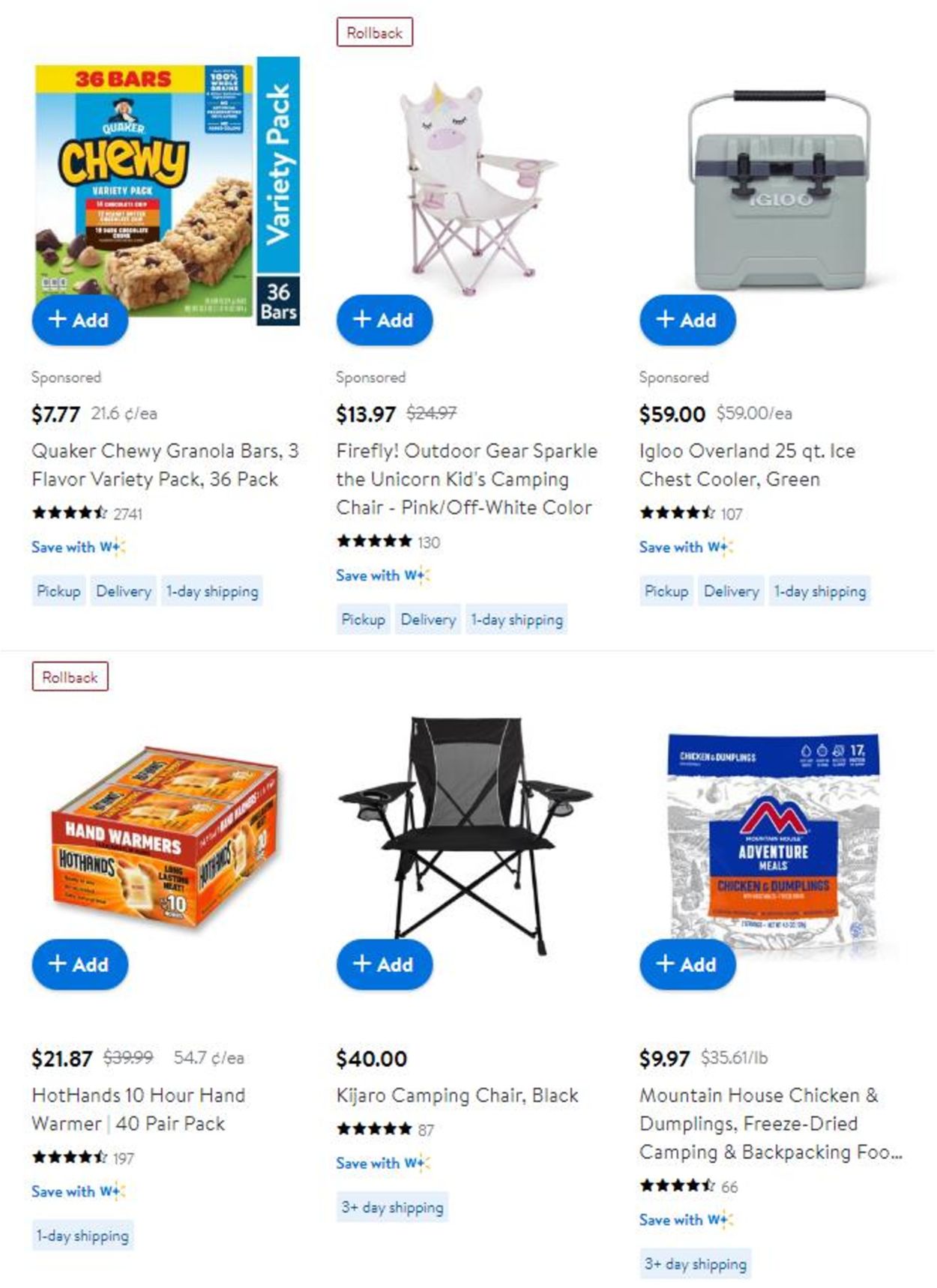The image is a vertically oriented screenshot showcasing various items available for purchase, arranged in two rows of three items each. The layout features a clean white background and includes detailed information about each product along with an "Add +" blue button for easy purchasing.

In the top row from left to right:
1. Quaker Chewy Granola Bars, 3 Flavor Variety Pack (36 Pack) - Priced at $7.77, rated 4.5 stars.
2. Firefly Outdoor Gear Sparkle the Unicorn Kids' Camping Chair (Pink/Off-White) - Priced at $13.97, rated 5 stars.
3. Igloo Overhead 25 Quart Ice Chest Cooler (Green) - Priced at $59.00, rated 4.5 stars.

In the bottom row from left to right:
1. HotHands 10 Hour Hand Warmer (40 Pair Pack) - Priced at $21.87, rated 4.5 stars.
2. KidJaro Champion Camping Chair (Black) - Priced at $40.00, rated 5 stars.
3. Mountain House Chicken and Dumplings Freeze-Dried Camping and Backpacking Food - Priced at $9.97, rated 4.5 stars.

Each product listing includes an image of the item, its name, price, customer rating, and the convenient "Add +" button to facilitate quick purchasing decisions.